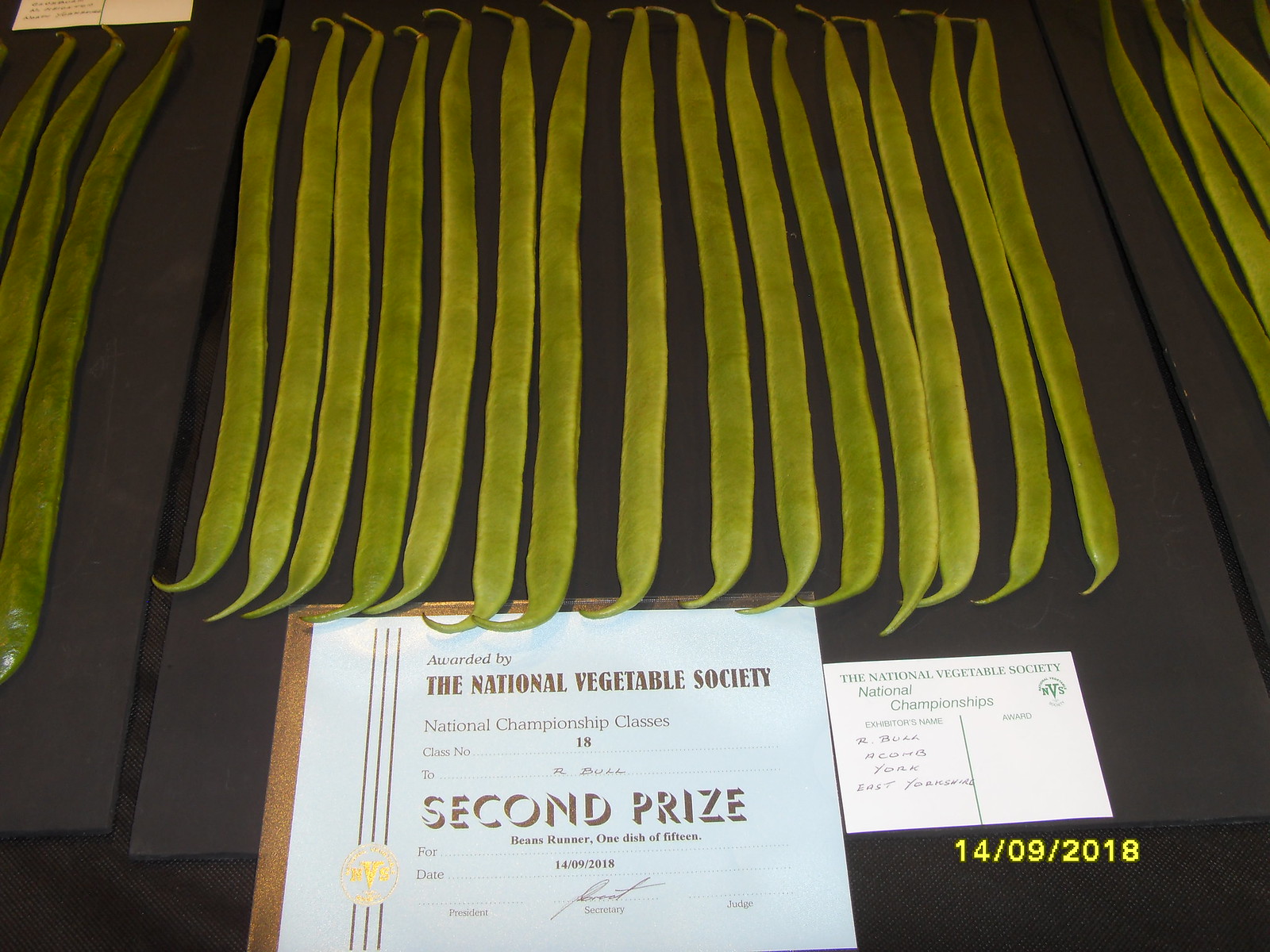This is a detailed photograph taken indoors of an award-winning display of vegetables, specifically runner beans. The focus is on a middle table, among three rows of beans, featuring a neatly arranged row of 17 long, green beans laid side by side on a black background. Below the beans is a notepad that bears the award details: it reads, "Awarded by the National Vegetable Society, National Championship Classes, Class Number 18." The award is designated as "Second Prize" in large font, with a handwritten note that mentions "R. Butt, Second Prize, Beans Runner, One Dish of 15." A timestamp in yellow font at the bottom right corner of the photograph indicates the date as "14-09-2018," which matches the smaller printed date on the notepad, affirming the award's authenticity. Another card to the right of the beans provides additional context, mentioning the National Vegetable Society's National Championships, although the text is less legible. The consistent details across all sources highlight the prize-winning status of these runner beans in the competitive arena of national vegetable displays.